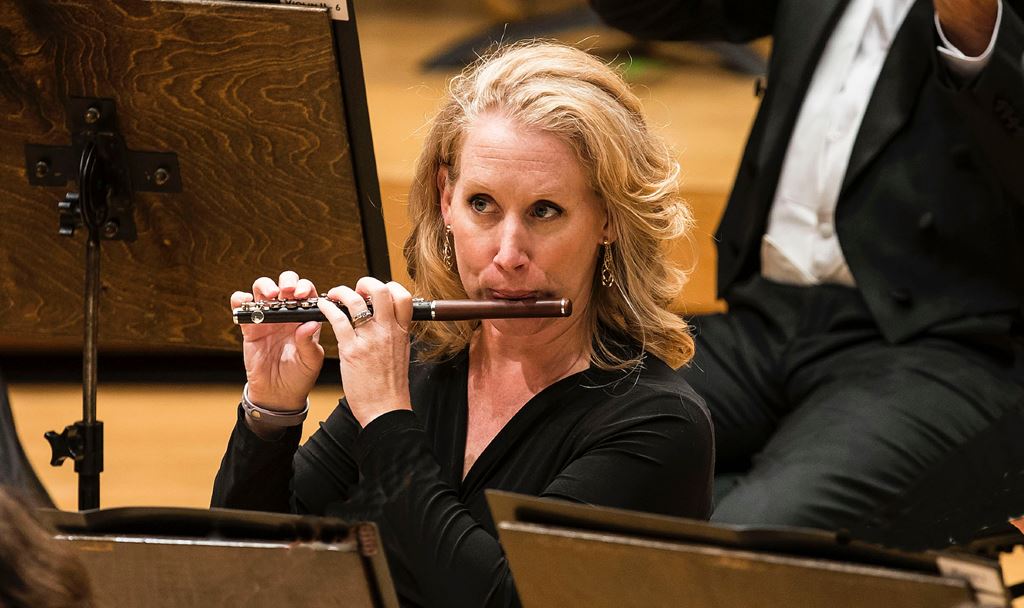In this photograph, we see a close-up of a professional flutist, positioned center stage during an orchestral performance. The flutist is a blonde-haired woman, likely in her 50s, with her hair slicked back. She wears earrings in both ears and is dressed in a solid black outfit. She holds a piccolo—its mouthpiece is brown while the main body is black—up to her lips, playing it with intense concentration.

Directly in front of her stands a music board with brown folders containing sheet music. The stage floor visible beneath her is a light beige wood. To her left, a microphone stand is partially visible. Behind her, slightly to the right, another musician is partially seen; based on the positioning of his arms, he is likely playing a violin. He is dressed in a formal black vested coat, white shirt, and black pants, typical attire for the orchestra. The backdrop of the stage emphasizes the structured elegance of the performance setting, further accentuating the focus and poise of the flutist.